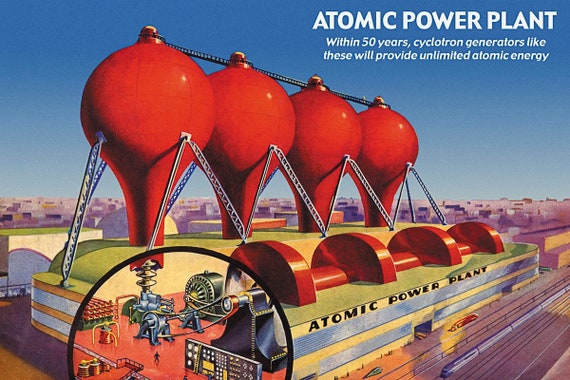This color illustration, set in a landscape orientation, depicts a retro-futuristic concept of an atomic power plant, styled with a science fiction flair. The upper right corner of the image features bold white text that reads "Atomic Power Plant," with smaller text beneath it stating, "Within 50 years, cyclotron generators like these will provide unlimited atomic energy," set against a blue sky background.

The central focus of the illustration is a large, two-story rectangular building with light yellow walls and a light green roof. The building has numerous windows and features "Atomic Power Plant" emblazoned in black text across the top. In front of the building, there are curved red metal pieces and a red pole.

Dominating the middle of the scene, four large, red spherical tanks—resembling either rubber balloons or upside-down onions—are elevated by tall ladders and connected by a black walkway. These tanks sit atop the building like industrial sculptures.

To the right of the structure runs a multi-lane highway, while the horizon is dotted with a city skyline, indicating the power plant's urban setting. Additionally, the bottom left corner includes a circular inset showing the detailed inner workings of the power plant, featuring computer boards and machinery, providing a glimpse into its advanced technology.